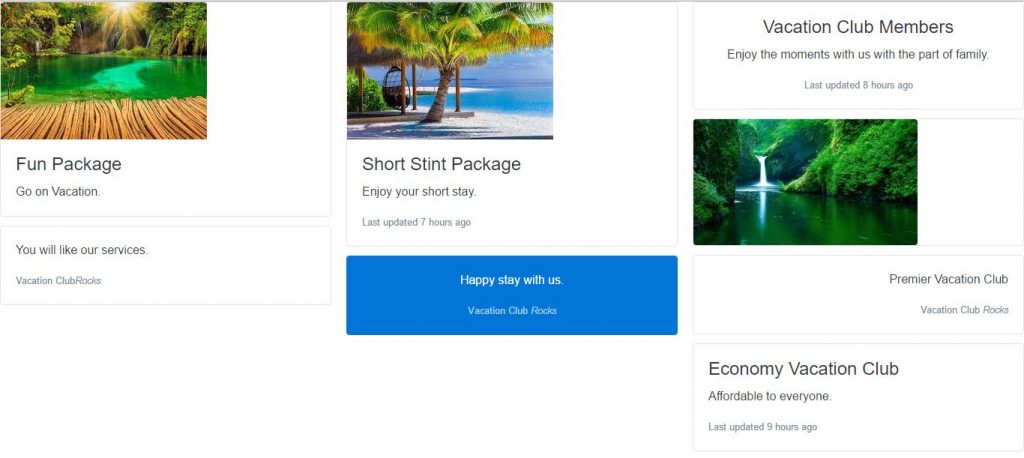A screenshot from a vacation website is displayed on a computer screen, divided into three main sections within a large rectangular layout.

**Left Section:**
- **Image:** In the upper left corner, there is an image depicting a serene green lagoon or lake, surrounded by lush trees. The atmosphere is tranquil, enhanced by the sunlight streaming down from the top. In the foreground, a wooden dock or path extends, inviting the viewer to imagine stepping into the scene.
- **Text Below Image:** "Fun Package"
- **Description:** "Go on vacation! You will like our services. Vacation Club rocks!"

**Center Section:**
- **Image:** Another image is placed in the upper left corner, showing a picturesque sandy beach. In the middle of the photo stands a palm tree, offering a typical tropical vibe. To the right of the tree, there is a hanging, egg-shaped chair, suggesting a spot for relaxation.
- **Text Below Image:** "Short Stint Package"
- **Description:** "Enjoy your stay."
- **Update Notice:** "Last updated seven hours ago."
- **Action Button:** Below this section, there's a large blue rectangle stating "Happy Stay With Us, Vacation Club Rocks," indicating an active or clickable button.

**Right Section:**
- **Image:** The upper left corner features an image of a breathtaking green body of water, with a cascade waterfall in the background, surrounded by dense trees on all sides, creating an idyllic natural setting.
- **Text Below Image:** "Vacation Club Members"
- **Description:** "Enjoy the moments with us. Be part of the family."
- **Update Notice:** "Last updated eight hours ago."
- **Additional Box:** Underneath, a smaller box highlights "Economy Vacation Club" with a tagline "Affordable to everyone," providing an update timestamp of nine hours ago.